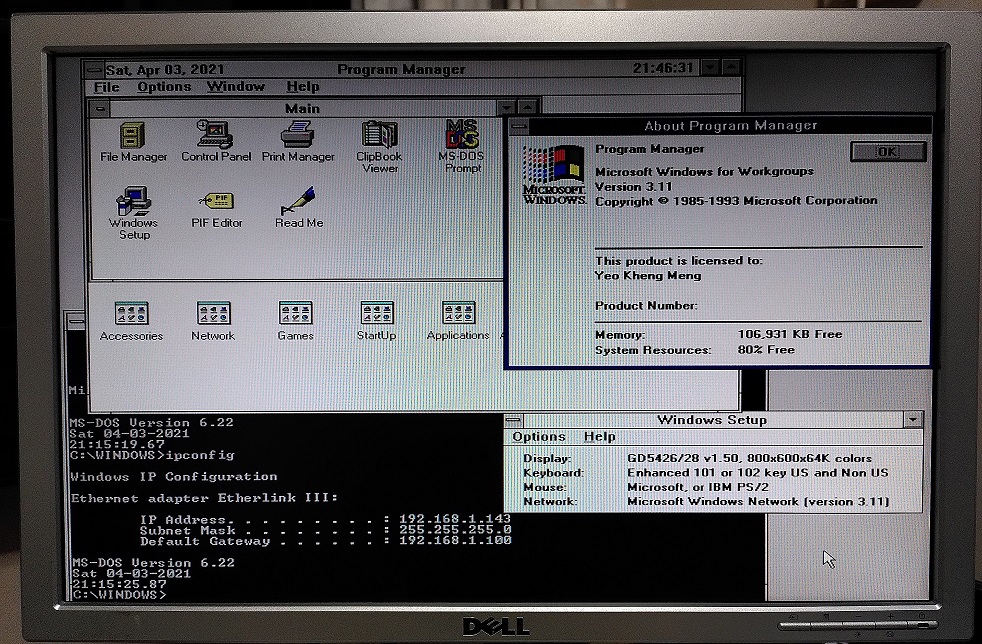The image depicts an old computer screen displaying Microsoft Windows for Workgroups Version 3.11, which was copyrighted between 1985 and 1993 by Microsoft Corporation. The main focus is on several windows open on the desktop. The Project Manager window is in the background, while the "About Project Manager" window is in the foreground with the Windows Setup window positioned below it. Another window, labeled Program Manager, displays various options including File Manager, Control Panel, Print Manager, and MS-DOS Prompt. Additional technical details are visible at the bottom, showing information like MS-DOS version 6.2, Windows IP Configuration, with IP addresses, subnet masks, and default gateways. The colors on the screen include yellow, blue, green, red, black, white, and gray. The outer border of the screen is silver. The interface prominently features the Microsoft Windows logo, reflecting the classic and iconic look of early Windows operating systems.